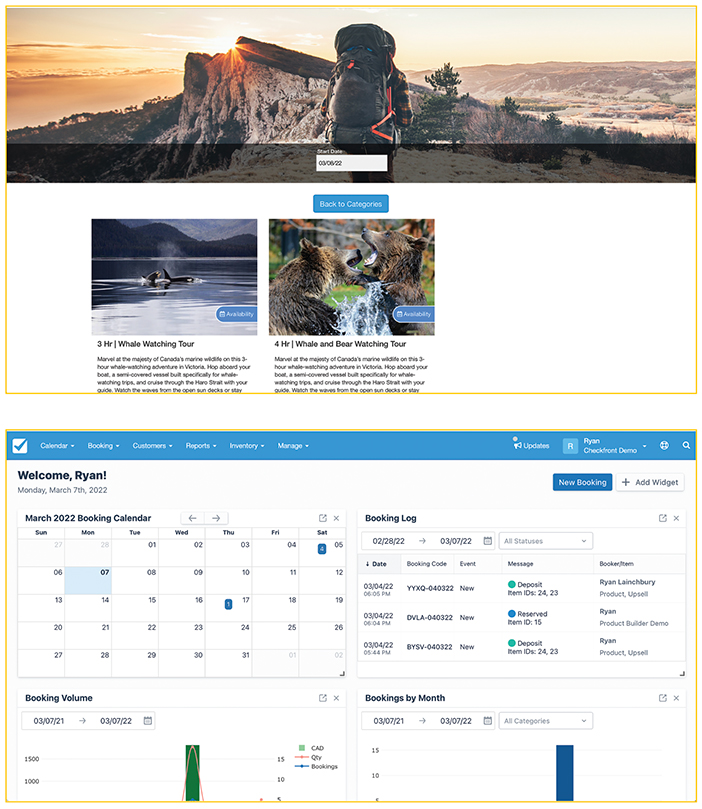At first glance, the webpage resembles a travel booking platform. The header showcases a captivating landscape image featuring a rugged mountain face adorned with trees. A lone hiker, equipped with a large backpack, is seen ascending towards the summit. A date field is conspicuously placed on this header, allowing users to input their desired travel date, though currently the displayed date appears somewhat unclear.

Upon entering a date, the website reveals a selection of suggested activities. The first option displays an image of orcas, advertising a "Three-Hour Whale-Watching Tour" with a brief description beneath it. Adjacent to this is another option, promoting a "Four-Hour Whale and Bear-Watching Tour" with its own description. Each activity image is accompanied by a clickable button featuring a calendar icon labeled "Check Availability."

Further down, the website offers personalized booking management for a user named Ryan. It welcomes him with a booking summary accompanied by a calendar and a log for current and past bookings. Ryan has the options to create new bookings and manage existing ones. The interface indicates his current bookings, highlighting a start date on the 5th of March and a notable booking on the 17th of March. This section solidifies the website’s function as a comprehensive travel management tool.